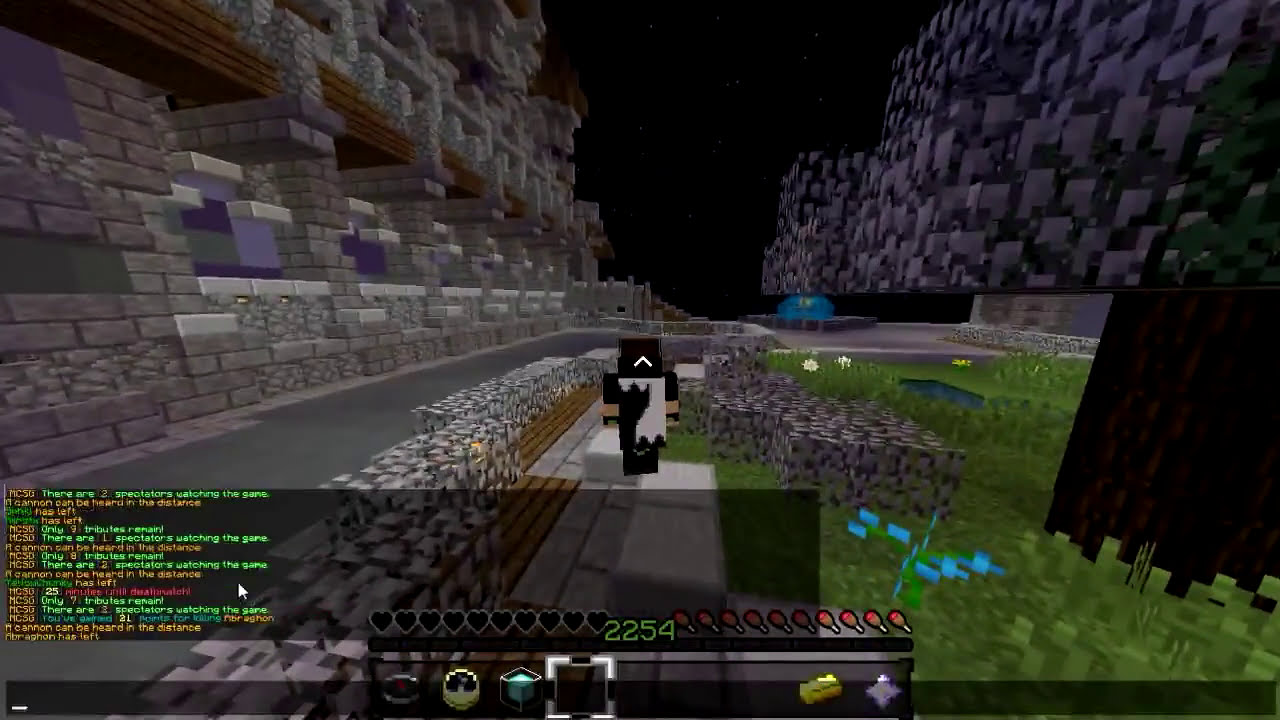The image is a screenshot from the video game Minecraft, characterized by its pixelated, blocky graphics. The setting is under a dark night sky dotted with small white stars. To the right, a rock wall floats above the ground, partially obscuring a brown tree trunk rooted in a field of green grass. Gray bricks dominate the midground, while a small black figure with a white front, resembling a knight in black armor with an upside-down V for a mouth, stands on light-colored concrete blocks. This figure, marked with some type of gray insignia on its chest, appears to be positioned in a courtyard bordered by two brick walls and intersected by zigzagging walkways and brick sidewalks. The left side of the scene features a large wall with shades of gray and purple. At the bottom left of the screen, a long gray chat box contains tiny, unreadable green, orange, and pink text. The center of the screen has a green number "2254" displayed, with a black bar underneath, and an array of game icons including hearts, porkchops, a compass, a clock, a beacon, a gold bar, and a diamond.